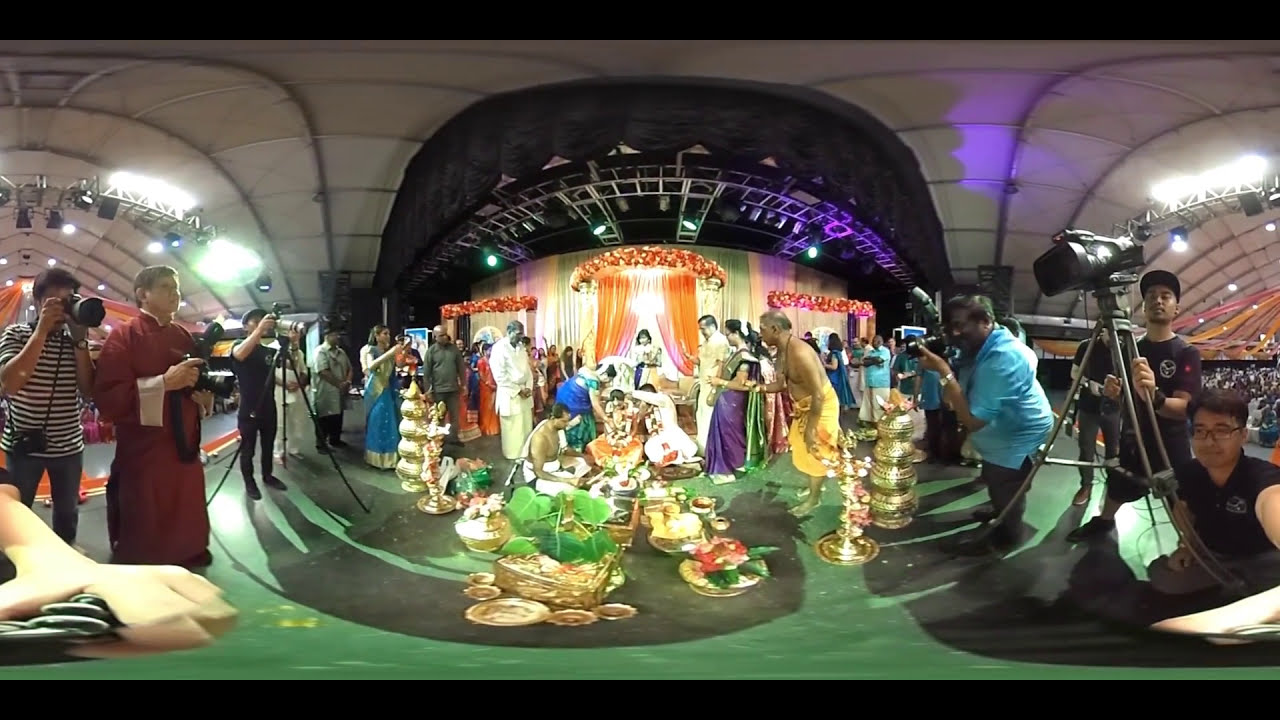The image depicts a vibrant and colorful indoor scene, possibly part of an event, ceremony, or TV set. The setting is inside a pavilion with a large white roof, featuring walls lined with bent silver or metal pipes that arch across the space. Centered prominently is a black arch adorned with silver-gray lines radiating outwards like a rainbow. Below the arch hangs a dazzling array of pastel curtains in shades of green, pink, and yellow, alongside bright orange drapes decorated with flowers.

On the green floor below, numerous brass or gold platters filled with food and green leaves are laid out, suggesting a ceremonial or festive context. The scene is bustling with people, some dressed in colorful clothing including long dresses in purple and green, while others wear white. A couple dressed in orange and white sits at the center, possibly indicating a wedding or significant ceremony, with various statues and golden-colored copperware around them.

The atmosphere is lively, with people on either side holding cameras and video equipment, capturing the event. The participants include individuals in black t-shirts, black and white stripes, and long dark red robes. The entire scene is framed by a stage-like setup, with an iron scaffolding above and a large light illuminating the area, complemented by striped curtains and fabrics in orange and yellow that create three archways. The combination of colorful decorations, ceremonial elements, and a crowd of onlookers contributes to the rich and festive ambiance of the scene.